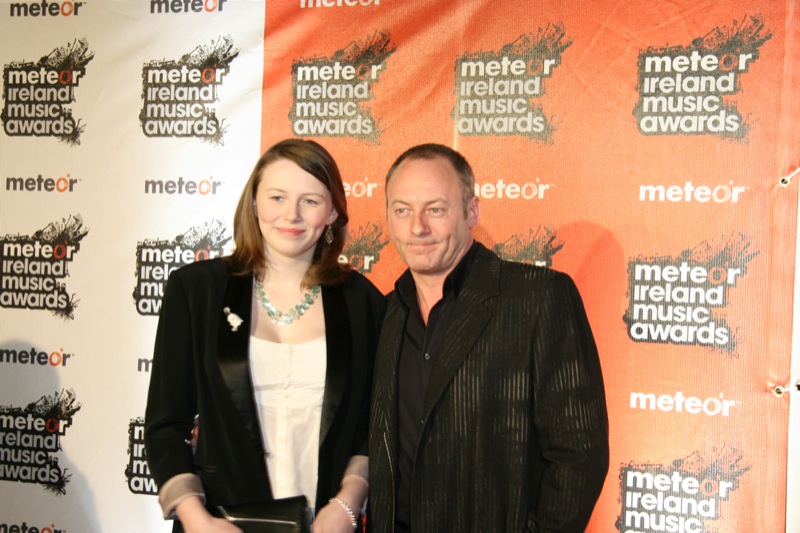In this color landscape photograph, taken at what appears to be a red carpet or press area for the Meteor Ireland Music Awards, two people stand prominently in front of a backdrop. The backdrop, which alternates between orange and white sections, features the event's logo repetitively, with the distinctive "Meteor" text containing an exploding "O."

On the left stands a white woman around 40 years old with shoulder-length brunette hair styled to the side. She is dressed in a black blazer, a white low-cut blouse, and wears a striking silver necklace. Her hands, holding a black purse, rest calmly in front of her waistline. To her right is a man, possibly an actor from Game of Thrones, aged around 45 with a receding hairline. He wears an eye-catching black suit jacket adorned with light face imprints, paired with a black button-down shirt. Both individuals are positioned centrally in the photograph, facing slightly towards the viewer, seemingly engaging with the press nearby.